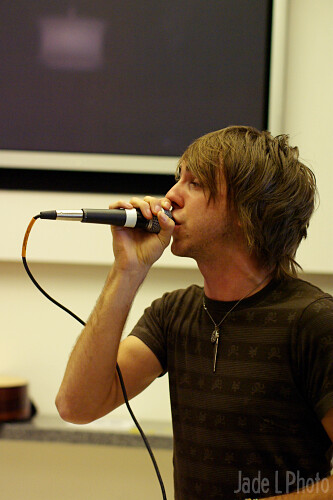This photo captures a young man deeply engaged in singing into a wired microphone, firmly pressed against his lips. He has a distinctive look with long, shaggy, light brown hair and some stubble on his face, reminiscent of an emo singer. His attire includes a dark brown shirt with horizontal light brown stripes and designs on the darker sections and a silver necklace. The background of the image features a blurry, nondescript room with a large, unwritten blackboard behind him. In the bottom right corner, a watermark reads "Jade L. Photo," indicating the photographer’s name. The photograph is taken at a vertical angle, emphasizing the intensity and focus of the young performer.